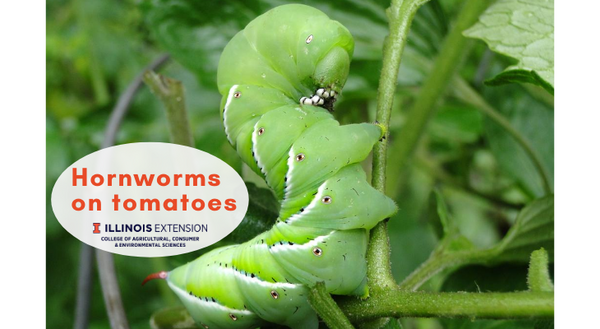The image features a vibrant, close-up shot of a neon green caterpillar, identified as a hornworm, clinging to a vivid green plant stem. The caterpillar's body exhibits a distinctive S-shape, with a head curved at the top and adorned with a small white eye and tiny white and black whiskers. Its surface is bulbous and marked by white stripes running along its sides, interspersed with small black dots. The caterpillar's chunky, almost spiral-like body also displays three short, triangular limbs with tiny fingers grasping the stem. An overlaid light gray oval on the left side of the image contains the red text "Hornworms on Tomatoes," and beneath it, in dark blue, reads "Illinois Extension, College of Agricultural, Consumer, and Environmental Sciences." The entire scene, including the out-of-focus green backdrop, evokes a fresh and natural ambiance.